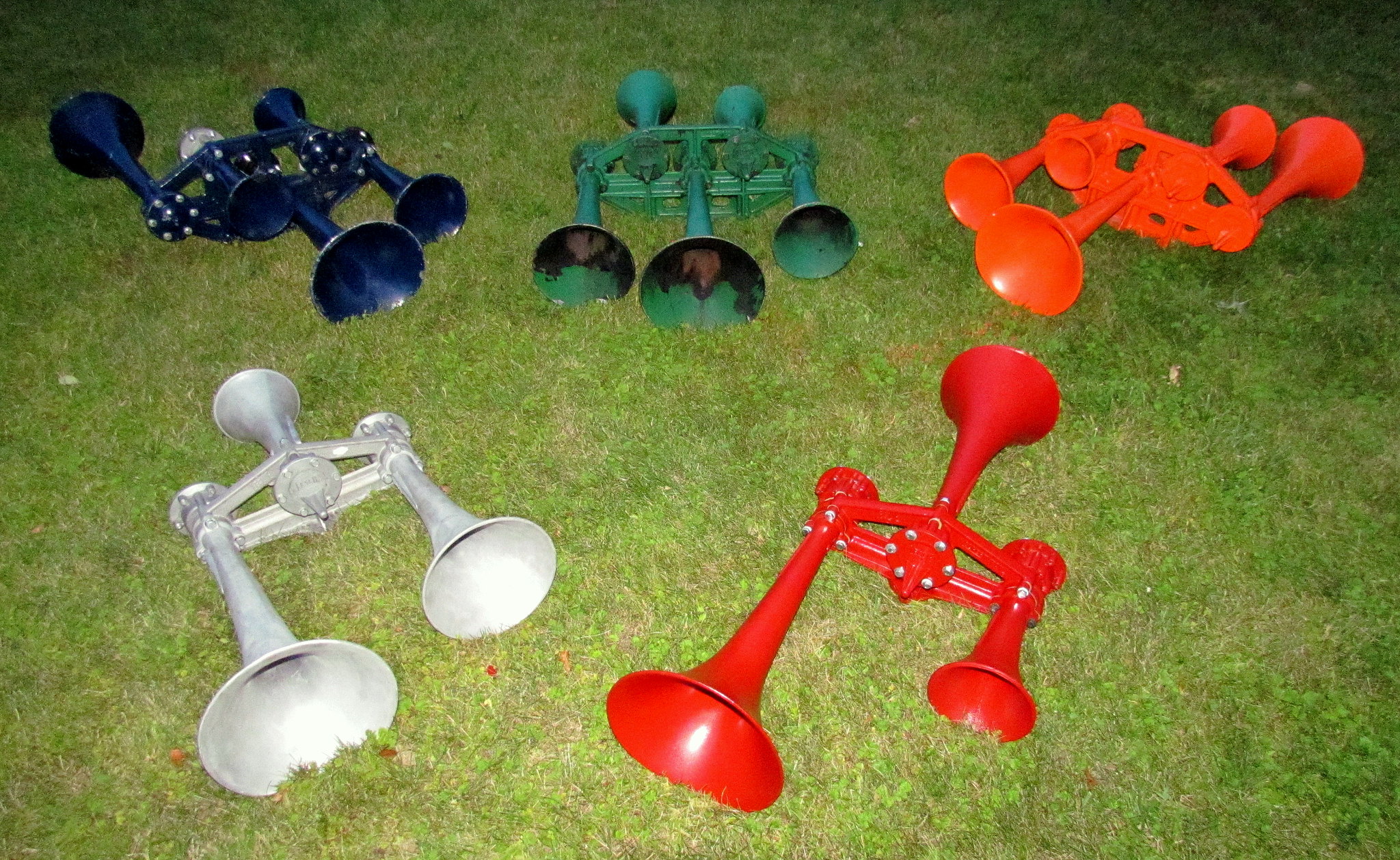The image displays five vibrant horn-like objects positioned on a lush expanse of bright green grass, captured in a landscape format. The horns are arranged with three in the top row and two in the bottom row. Each horn assembly features between three and five individual horn components of varying sizes, attached to a central bracket. 

In the top row, the leftmost item is dark blue with silver hardware, flaunting three horns on one side and two on the other. The central item is lime green, similarly configured with three horns on one side and two on the other. Completing the top row, the item on the right is a striking highlighter orange, also with three horns on one side and two on the other.

The bottom row presents a silver item on the left, which possesses two horns on one side and one on the other, and a vivid red item on the right with an opposite configuration of one horn on one side and two on the other. The harmonious color arrangement and the distinctive horn structures make this a fascinating and visually engaging composition.